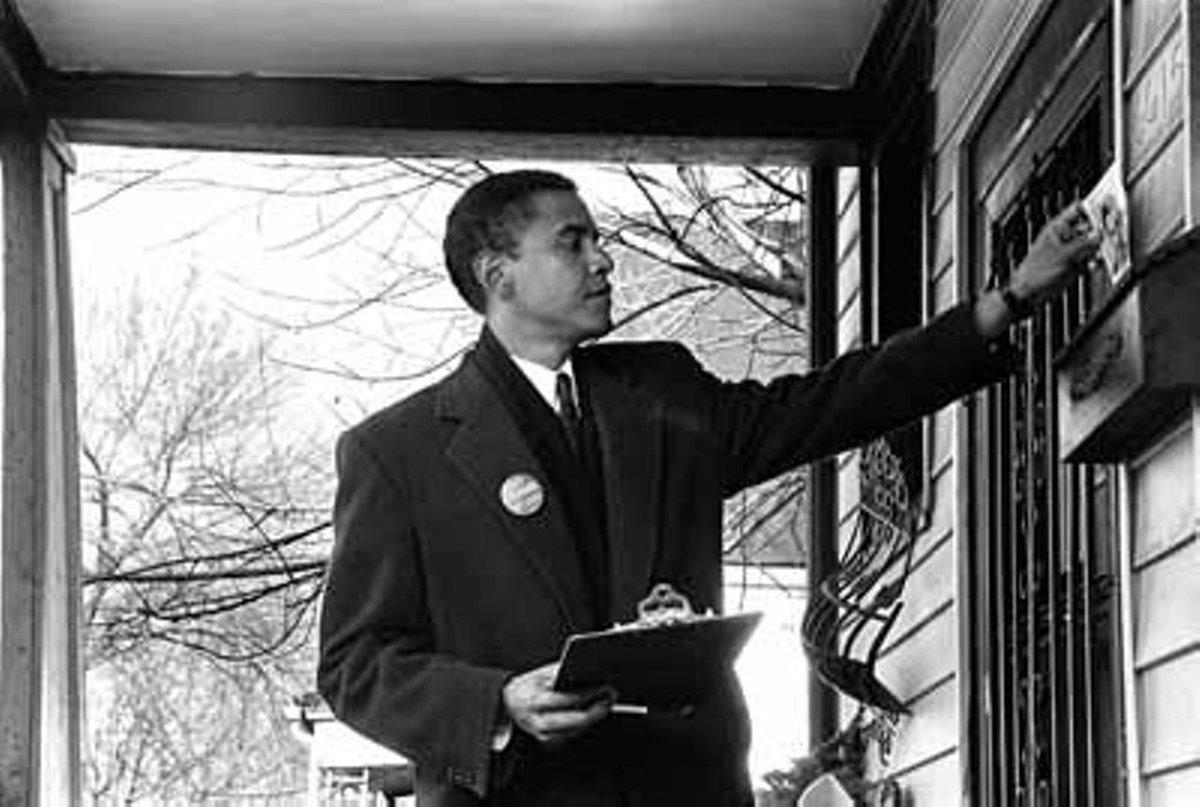In this black and white photo, former President Barack Obama is depicted in a black overcoat over a suit, complete with a white shirt, black tie, and a pin on the left side of his jacket. He stands on the porch of a house with siding and a railing, surrounded by trees under a pale sky. Obama appears to be engaged in political canvassing, evidenced by the clipboard in his right hand and the pamphlet or flyer he is placing into a mailbox attached to the house. His demeanor is focused as he performs this door-to-door activity, likely seeking voter support.